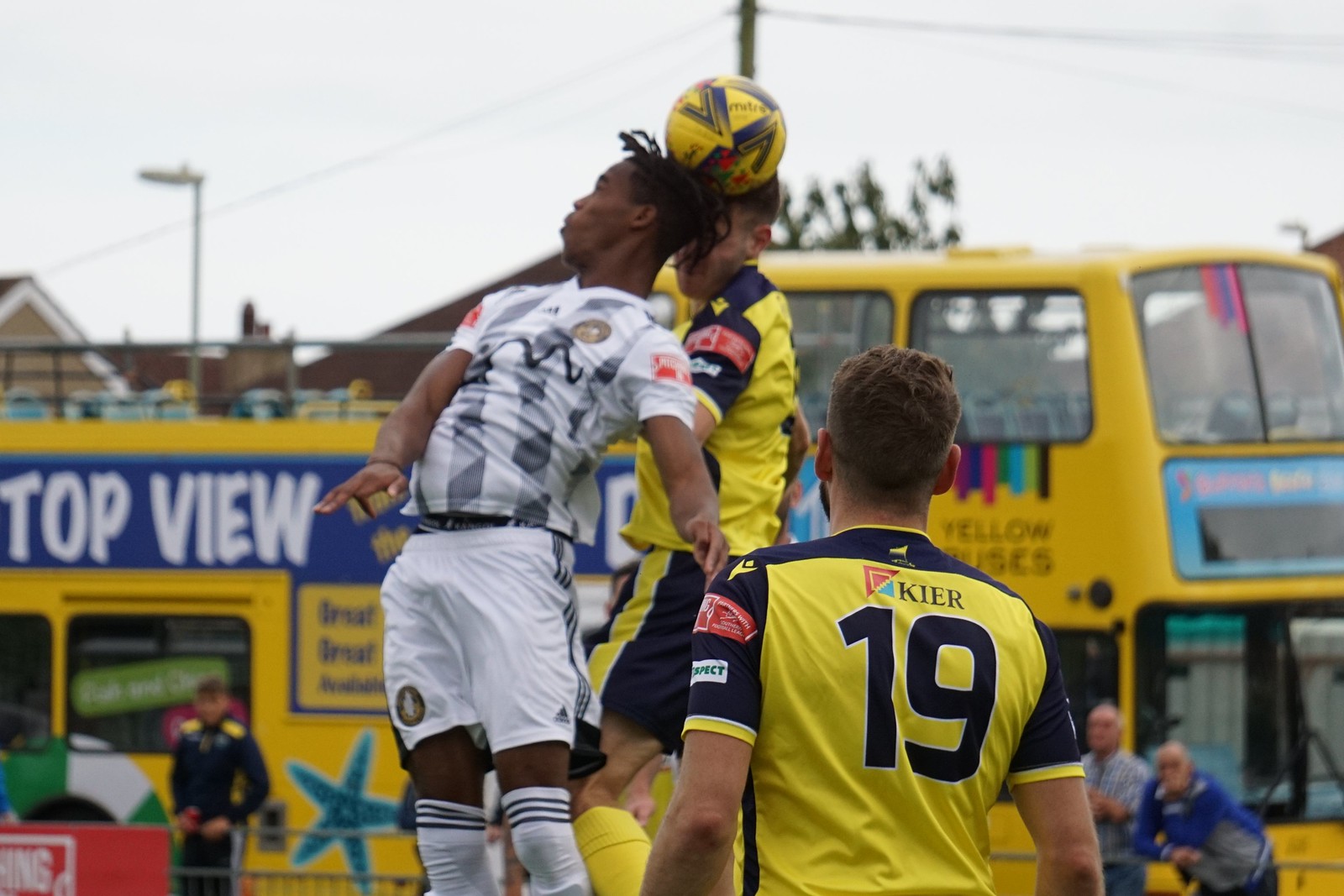In this photorealistic image, a dramatic moment from a soccer game is captured. At the center, an African player with dark skin and braided hair is mid-jump, his arms extended on either side as he heads a yellow and navy soccer ball. He wears a white and gray patterned jersey with red accents on the shoulders, paired with white shorts and socks. Right behind him, an opposing player, whose face is obscured, also leaps towards the ball. This player is dressed in a red and navy jersey with matching pants and yellow socks. In the foreground stands another player from the red and navy team, turning away from the camera. He has short brown hair and sports the number 19 in black on the back of his jersey. The background reveals a crowd of spectators leaning against a distant fence, slightly out of focus, and a bright yellow double-decker tourist bus with "Top View" written in white text on a blue banner on its side. The sky overhead is dark and gray, adding to the intensity of the scene.